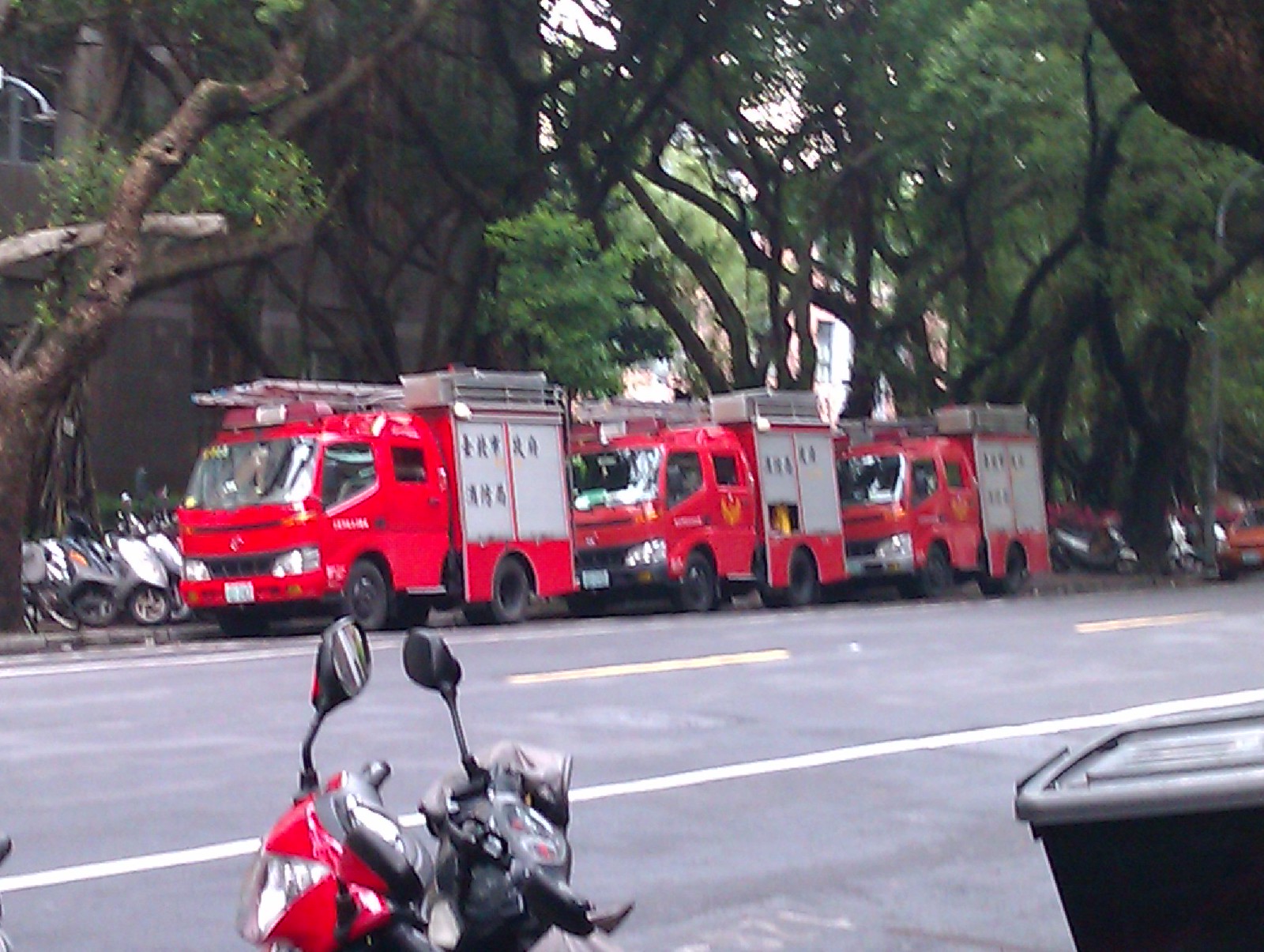This daytime photograph captures a bustling city street scene. In the foreground, a red motorcycle and a black trash can are visible, marking the image's lower portion. The street is divided by a white line, with yellow lines also present closer to the camera. The background features a row of small red firetrucks, adorned with silver ladders and Chinese characters on their sides, parked one behind the other on the left side of the road. To the left of the firetrucks, several silver mopeds are parked on the sidewalk. Behind these vehicles, verdant trees with twisting branches and dense foliage line the street, partially obscuring a mix of dark and light buildings in the distance. A sliver of sky peeks through the treetops, adding depth to the urban landscape. Farther to the right, behind a tree, the outline of a red car, possibly a sports car, is faintly visible.